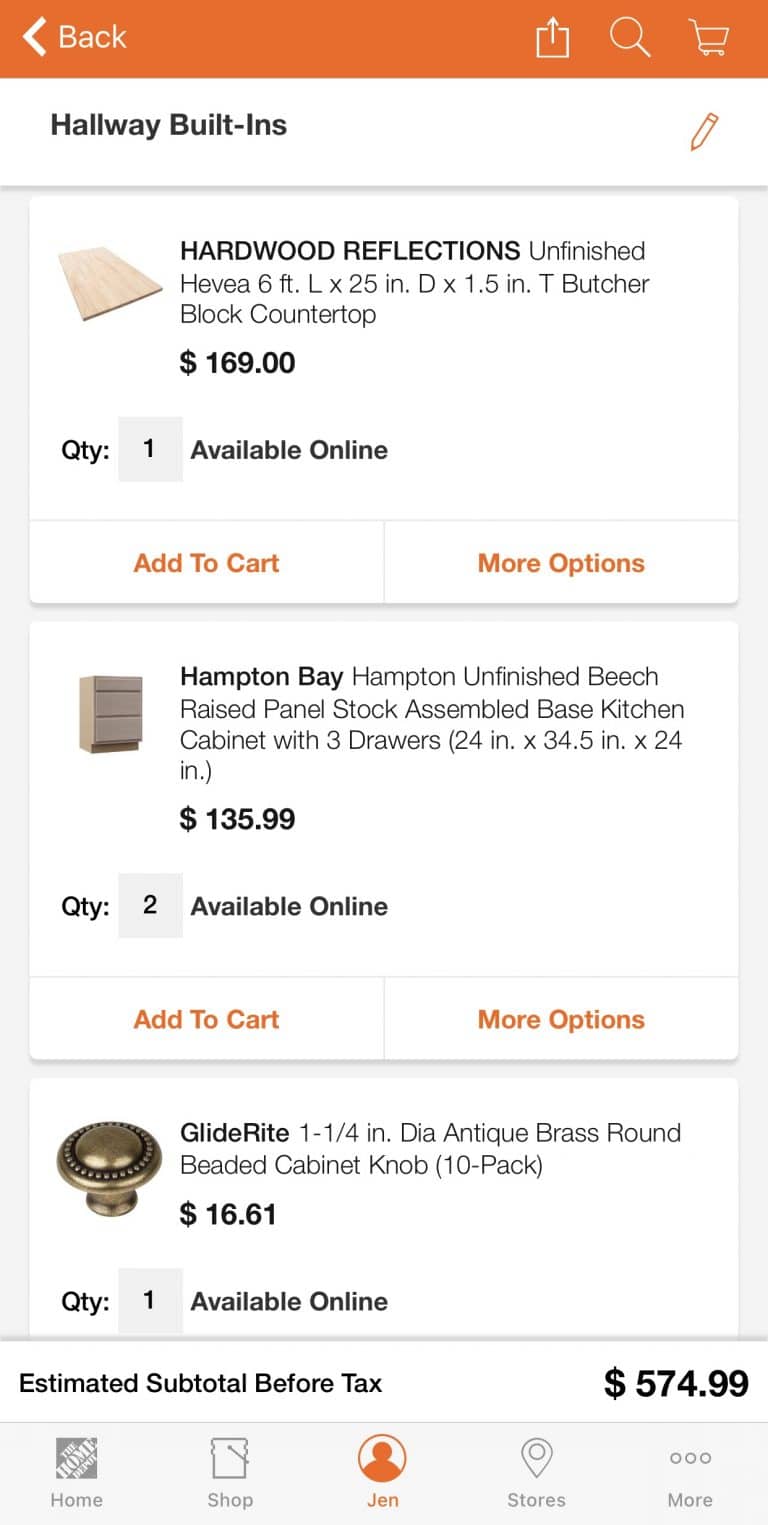In the image, we see a detailed screenshot showcasing various materials available for purchase that can be used in renovation projects, such as for the kitchen or garage. The items listed appear to be cabinetry and other related products, potentially for a hallway built-in. 

At the top of the list is a "Hardwood Reflections Unfinished Butcher Block Countertop," measuring 6 feet by 25 inches. This countertop, priced at $169 USD, is available online and can be added to the cart. The screenshot shows a user-made selection, indicating an online purchase option.

Below the countertop, we see the "Hampton Bay Unfinished Beach Raised Panel Stock Assembled Base Kitchen Cabinet," which features three drawers. This cabinet is priced at $135.99 USD, with two units available for online purchase and an option to add to the cart as well.

Further down, the image displays the "Glide-Rite 1/4 inch Antique Round Brass Beaded Cabinet Knob." These cabinet pulls, priced at $16.61 USD each, can be used with the aforementioned Hampton Bay cabinet. Only one of these knobs is available for online purchase. 

The grand total for these selected items - the butcher block countertop, the Hampton Bay cabinet, and the cabinet pulls - sums up to $574.99 USD. Overall, the screenshot indicates an online shopping scenario for cabinetry and hardware, likely intended for a kitchen, garage, or hallway renovation project.